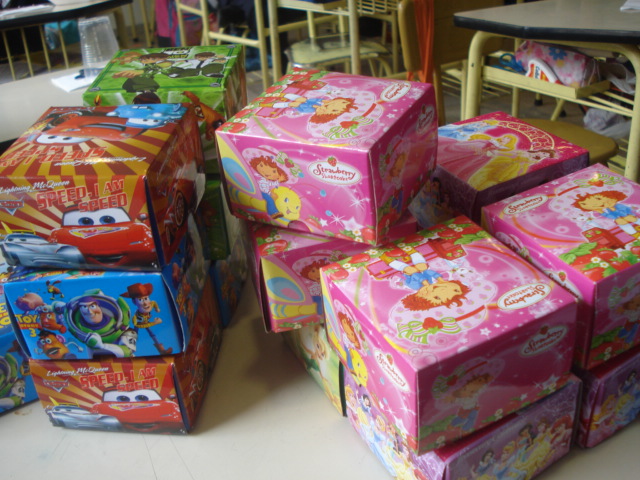This detailed image depicts a variety of children's toy boxes arranged in a classroom-like setting with tables and desks in the background. On the left side of the image, there are distinctive pink boxes featuring Strawberry Shortcake, which prominently display a girl with red hair and a pink hat, riding a yellow butterfly. Her name, "Strawberry Shortcake," is written in white letters against a cream-colored outline. 

To the right of these are stacks of toy boxes related to popular movie characters. The bottom left corner reveals a box labeled "Speed Jam" showcasing a red car with black, white, and dark red eyes. Positioned above it is a blue box featuring characters from Toy Story 3: Woody the cowboy, Buzz Lightyear the astronaut in a light green suit, and Mr. Potato Head, all set against a blue background. 

In front of these, there's another stack of similar "Speed Jam" boxes, again displaying red cars. Additionally, there's a small green action figure box with a child striking a running pose. The classroom setting includes tables with yellow metal curved legs and yellow shelves in the background, devoid of any children, emphasizing the arrangement of about sixteen various pink Strawberry Shortcake and other toy boxes in an educational environment.